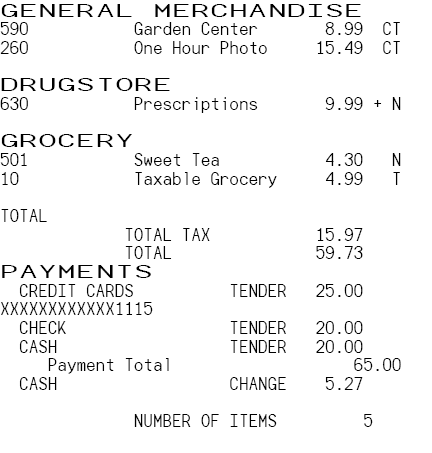The image shows a detailed receipt characterized by basic black text on a white background, listing the purchase information and payment details. The top of the receipt indicates several categories and items: General Merchandise, including 590 from the Garden Center priced at $8.99 and 260 from the One Hour Photo section at $15.49, both marked with "CT." In the Drugstore section, item 630 for Prescriptions priced at $9.99 is noted with "plus N." Moving to the Grocery section, item 501 is Sweet Tea for $4.30 labeled "N," and item 10 is Taxable Grocery for $4.99 marked "T." The total tax amount is $15.97, leading to an overall total of $59.73. Payment breakdown shows a credit card payment of $25 (last four digits 115), a check payment of $20, and a cash payment of $20, summing up to $65, hence a change of $5.27. The receipt also lists the number of items purchased as 5.